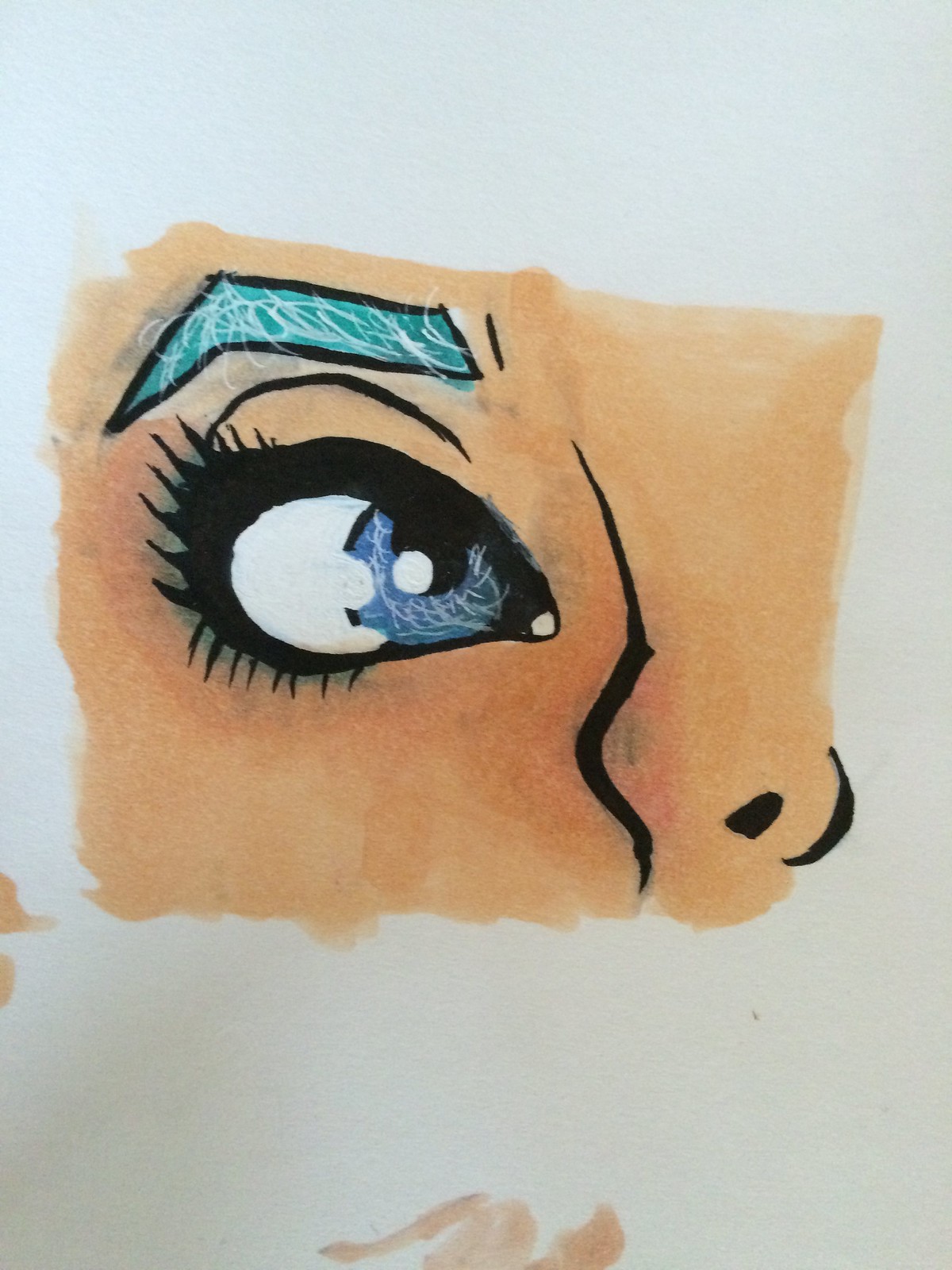This artwork is rendered on a piece of white paper, depicting an evocative portion of a face centrally framed within a rectangular section. The background showcases a skin tone, with the artwork focusing on intricate facial details. On the right-hand side of the image, approximately an inch from the paper's edge, a delicately drawn black outline forms the partial view of a nose. Just above this, a boldly colored, thick eyebrow stands out, filled with a vibrant blue hue interspersed with white squiggles, all meticulously outlined in black. 

The large, expressive eye is accentuated with dramatic black makeup and mascara, drawing attention to its intense detail. Within the eye, the white of the sclera is visible, and just to the left sits a striking blue circle decorated with white squiggles. A segment of this blue circle is intriguingly cut out, and nestled within it is a white pupil, adding depth and intrigue to the gaze.

Beneath this captivating portion of the face, slight remnants of the flush-colored paint used to create this artwork trail off towards the bottom and right side of the composition, suggesting the artist’s meticulous process and adding a touch of raw, creative authenticity.